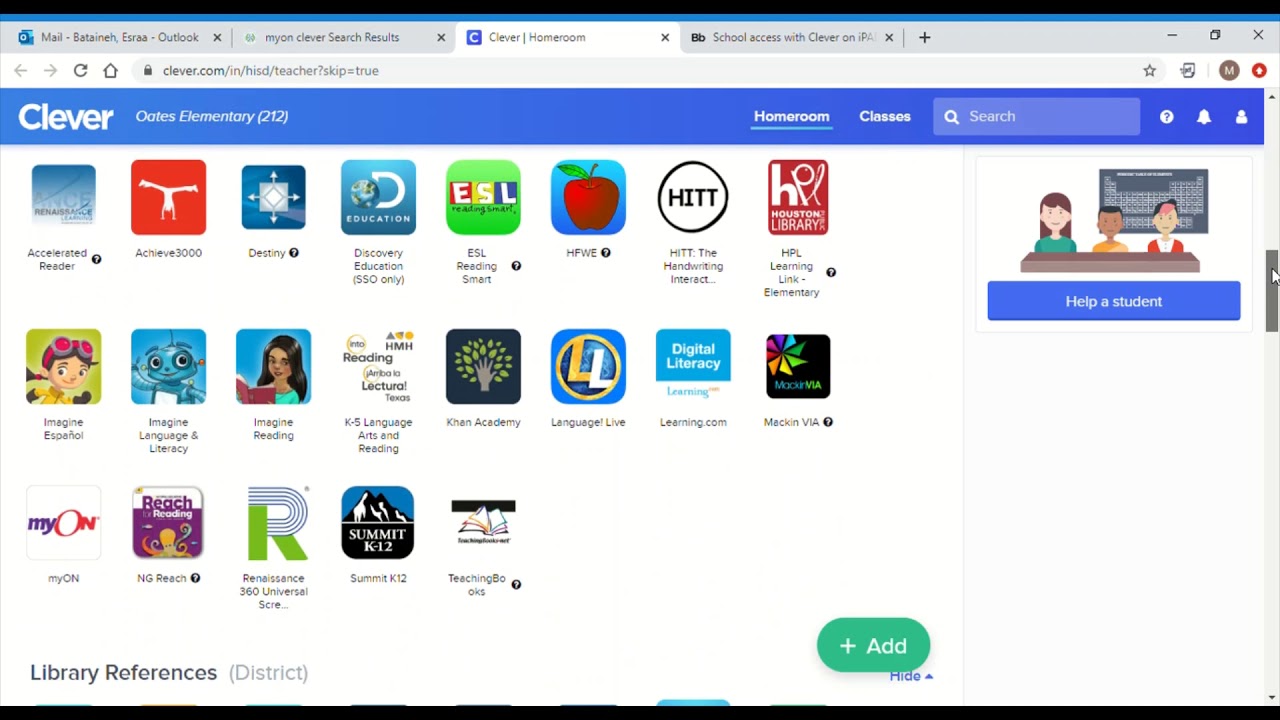In this image, we see a screenshot of a Windows interface. The open application is a Google Chrome web browser displaying several tabs. From left to right, the tabs include: Outlook Mail, a "My on Clever" search results page, the currently active "Clever Homeroom" tab, a "School Access with Clever on iPad" tab, and the Clever website. 

The address bar shows the URL for the Clever website, and the top-left corner features the Clever logo alongside the label "Oats Elementary 212 Homeroom." Below, various educational resources are listed as tabs, including Accelerated Reader, Achieve 3000, Destiny, Discovery Education, ESL Reading Smart, Imagine Español, and Language Live.

On the right side of the webpage, there is a search bar, a notification bell icon, and a "Help a Student" tab, all located in the top-right corner of the screen.